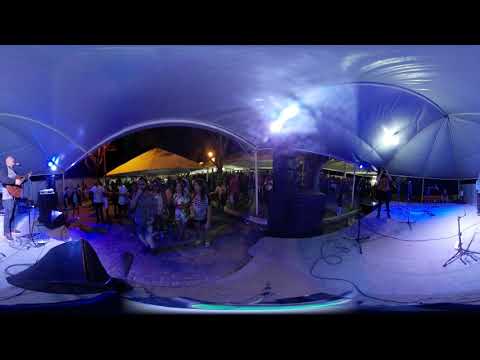This photograph captures the lively scene inside a blue-roofed tent set against the backdrop of a dark, nighttime sky. The focal point is a musician, likely a guitarist and singer, positioned to the left with a microphone stand beside him. This musician is actively playing music for the assembled crowd. The audience within the tent appears to be standing, enjoying the music, while some might be seated on picnic benches. Illuminating the scene are several neon LED lights and horizontal black strips that add to the ambiance.

Surrounding this central tent is an outdoor area visible through its entrances, where more people have gathered. This exterior space features additional tents, suggesting a festival or concert setting with various activities or shops around. The ground appears to be covered in snow, adding to the wintery atmosphere. Altogether, the image presents a vivid depiction of a musical event full of energy, with a bluish color theme dominating the top and contrasting with the darker elements below.